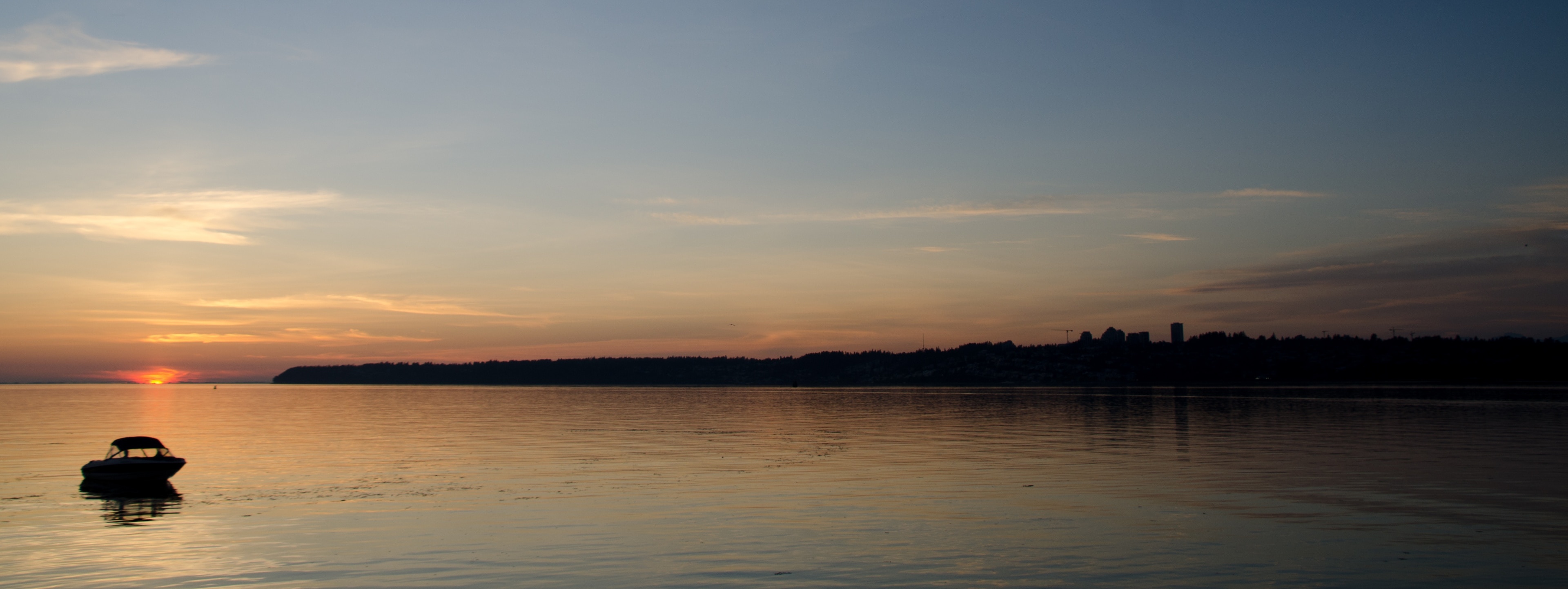This panoramic photograph captures a serene lake at either sunset or sunrise, showcasing a symphony of colors that transition from dark pink, oranges, and yellows at the horizon to light and dark blues higher up in the sky, punctuated by white clouds. The glowing orange sun appears to almost touch the water's surface, casting a warm reflection on the lake, particularly illuminating the left side. In the water, slightly left of center under the sun’s reflection, sits a small motorboat, its silhouette striking against the peaceful, still waters. The far distance reveals a tree-lined shore or island, spanning the entire width of the image, appearing as a dark, shadowy mass. The overall ambiance is one of tranquility and natural beauty, with the scene growing darker towards the right, reinforcing the calmness of dusk or dawn.